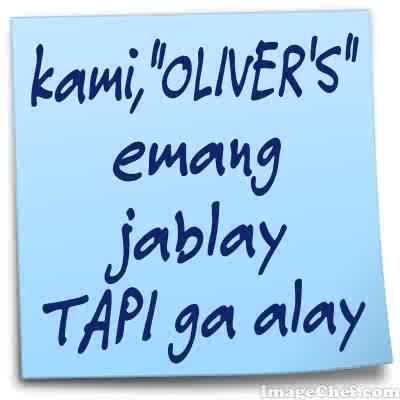The image depicts a digital representation resembling a light blue post-it note positioned slightly crooked in the center of a solid white background. The note features dark blue text written in a different language, organized in four lines. The text reads: "Kami, Oliver's," followed by "Eemang," "Jablay," and "Tapi Gah Olay." The watermark, "imagechef.com," is located in the bottom right corner. The overall visual effect includes some shading at the bottom of the note, suggesting a three-dimensional quality typical of a stock image, potentially indicating a copyrighted work.